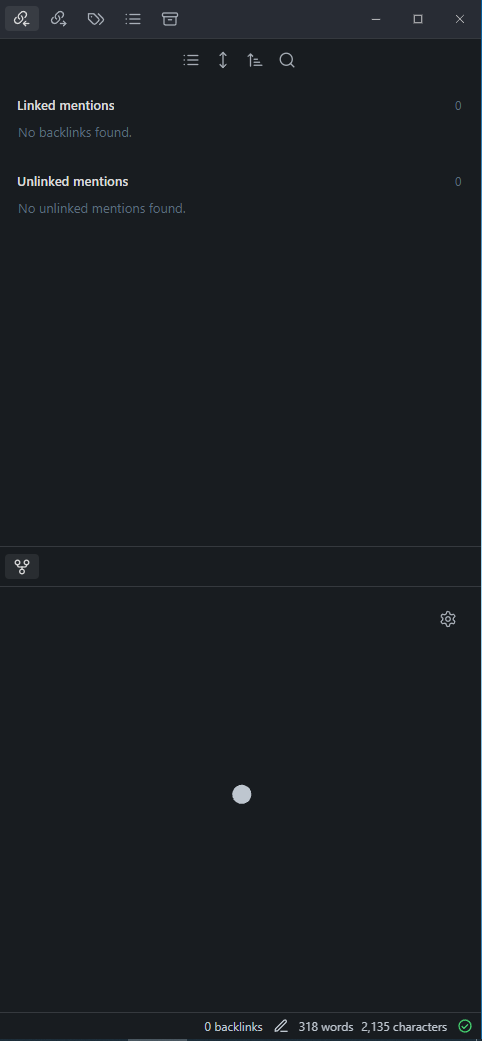The image portrays a screenshot of an application interface on a phone, characterized by an abundance of blank black space, creating a somewhat disconcerting and minimalist aesthetic. The layout is divided into two main sections or panels: a top panel labeled "Linked Mentions" and "Unlinked Mentions," suggesting a possible connection to social media tracking, perhaps Twitter, although no specific links or information are displayed. The top section features several icons, including chain links and labels, and what appears to be a trash or box icon, though their functions are not clear. The bottom panel is similarly empty, featuring a settings gear icon in the top-right corner. At the very bottom of the screen, numerical indicators read: zero backlinks, 318 words, and 2135 characters, though these numbers seem disjointed from the rest of the content, as no textual or character data is visibly present. The overall feel is reminiscent of coding software, with its segmented spaces and plethora of unused area.